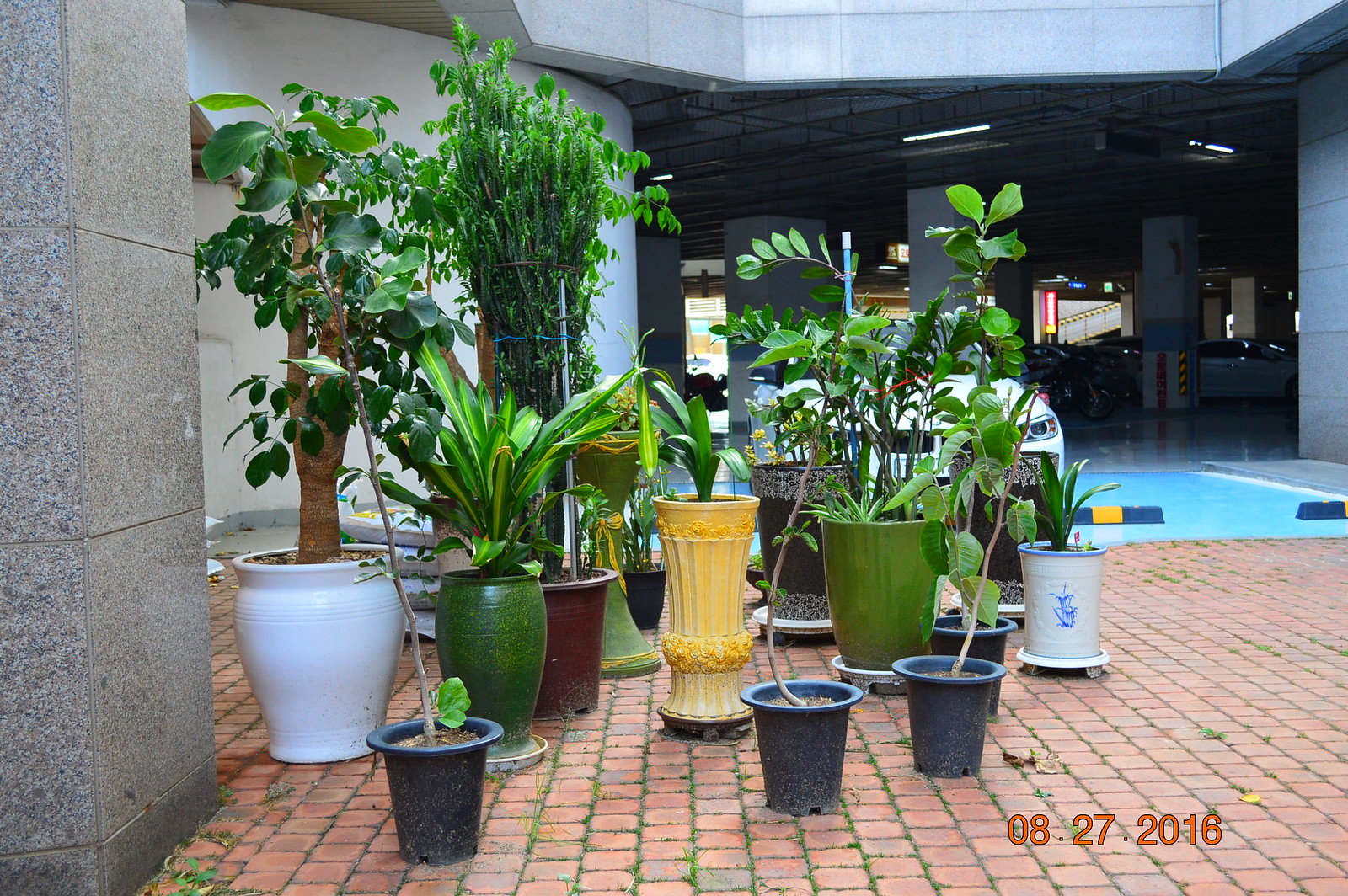The photograph, dated August 27, 2016, captures a diverse arrangement of potted plants positioned on a red brick pavement, speckled with light green moss. These plants, anchored in a mix of large and small pots, are carefully situated in front of what appears to be a large building or parking garage, evident from the concrete pillars and dimly lit parking spaces in the background. A white BMW, partially obscured by the plants, is parked just behind them, highlighting the urban setting.

Starting from the foreground, three round black pots hold tall plants with green leaves. Behind these, a large white porcelain pot houses a tree-like plant with a sturdy trunk. Adjacent to it, a light green pot, a distinctive bright yellow pot with vertical lines, and another lighter green pot each support their own lush greenery. To the right, a white pot with blue rims and a blue decorative image contains additional foliage. A reddish pot in the background, secured with string and a supporting pole, stabilizes its lofty plant. The left side features a prominent concrete pillar, anchoring the scene to the architectural environment. The intricate details of the pots—from colors to structural supports—highlight the careful cultivation and aesthetic arrangement of the garden in this urban oasis.